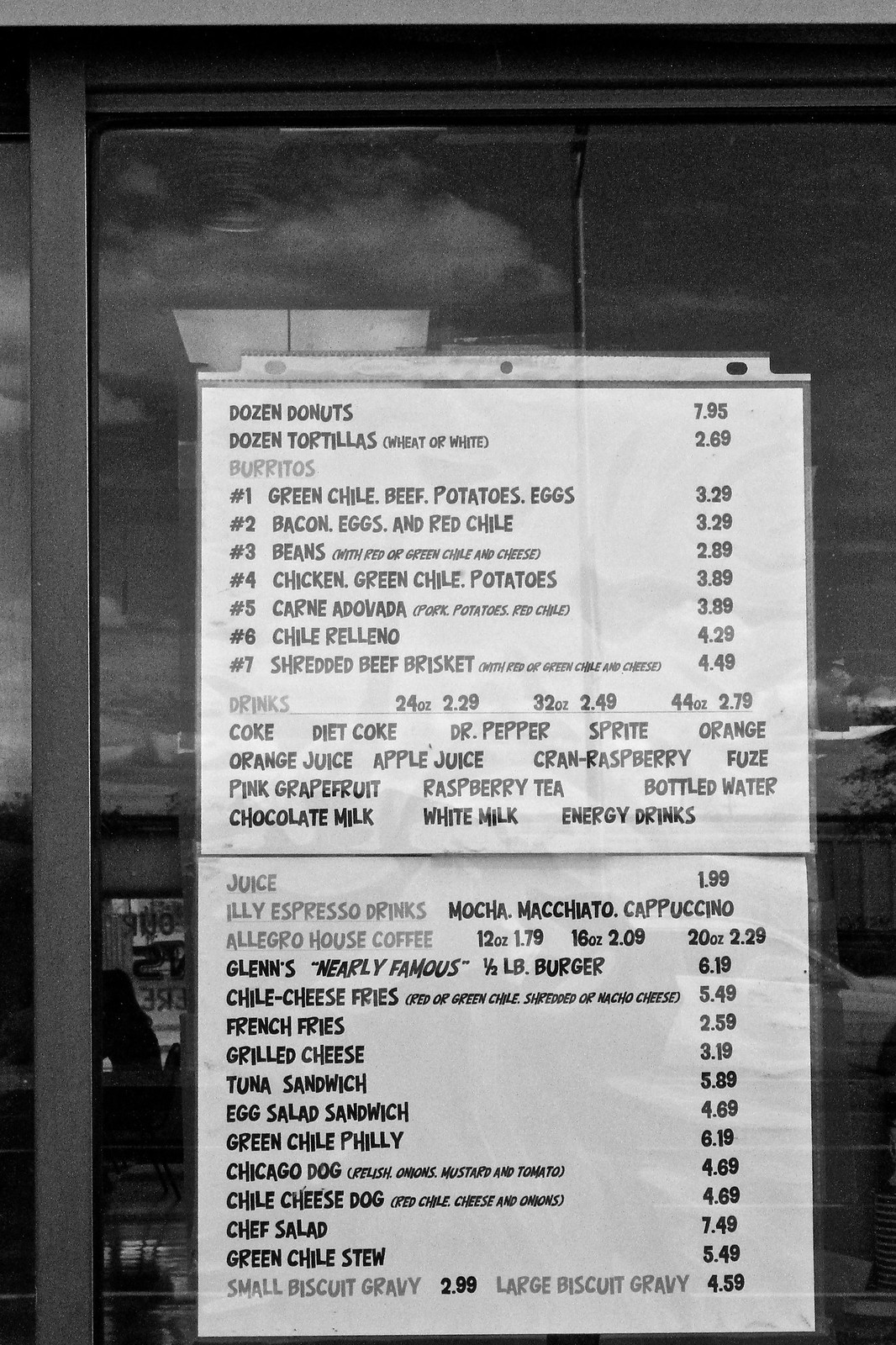The image showcases a restaurant menu, meticulously enclosed in a protective binder sleeve and securely taped to the front of a window or door, shielding it from rain or water. The menu, written predominantly in black text with certain headings and items highlighted in gray, offers a diverse selection of foods and beverages:

**Doughnuts & Tortillas:**
- Dozen Doughnuts: $7.95
- Dozen Tortillas (Wheat or White): $2.69

**Burritos:**
- #1 Green Chili, Beef, Potato, and Eggs: $3.29
- #2 Bacon, Eggs, and Red Chili: $3.29
- #3 Beans with Red or Green Chili and Cheese: $2.89
- #4 Chicken, Green Chili, and Potatoes: $3.89
- #5 Carne Adovada (Pork, Rice, and Red Chili or Pork, Potatoes, and Red Chili): $3.89
- #6 Chili Relleno: $4.29
- #7 Shredded Beef Brisket with Red or Green Chili and Cheese: $4.49

**Drinks:**
- 24 ounces: $2.29
- 32 ounces: $2.49
- 44 ounces: $2.79
- Options: Coke, Diet Coke, Dr. Pepper, Sprite, Orange, Orange Juice, Apple Juice, Cran-Raspberry, Fuze, Pink Grapefruit, Raspberry Tea, Bottled Water, Chocolate Milk, White Milk, Energy Drinks

**Specialty Drinks:**
- Juice: $1.99
- Illy Espresso Drinks (Mocha, Macchiato, Cappuccino)
- Allegro House Coffees:
  - 12 ounces: $1.79
  - 16 ounces: $2.09
  - 20 ounces: $2.29

**Main Dishes & Snacks:**
- Glenn’s Nearly Famous Half-Pound Burger: $6.19
- Chili Cheese Fries (Red or Green Chili with Shredded or Nacho Cheese): $5.49
- French Fries: $2.59
- Grilled Cheese: $3.19
- Tuna Sandwich: $5.89
- Egg Salad Sandwich: $4.69
- Green Chili Philly: $6.19
- Chicago Dog (Relish, Onions, Mustard, Tomato): $4.69
- Chili Cheese Dog (Red Chili, Cheese, Onions): $4.69
- Chef Salad: $7.49
- Green Chili Stew: $5.49
- Biscuit & Gravy:
  - Small: $2.99
  - Large: $4.59

The entire menu is presented in a clear, organized manner, with specific sections and items distinctly marked for easy reading.